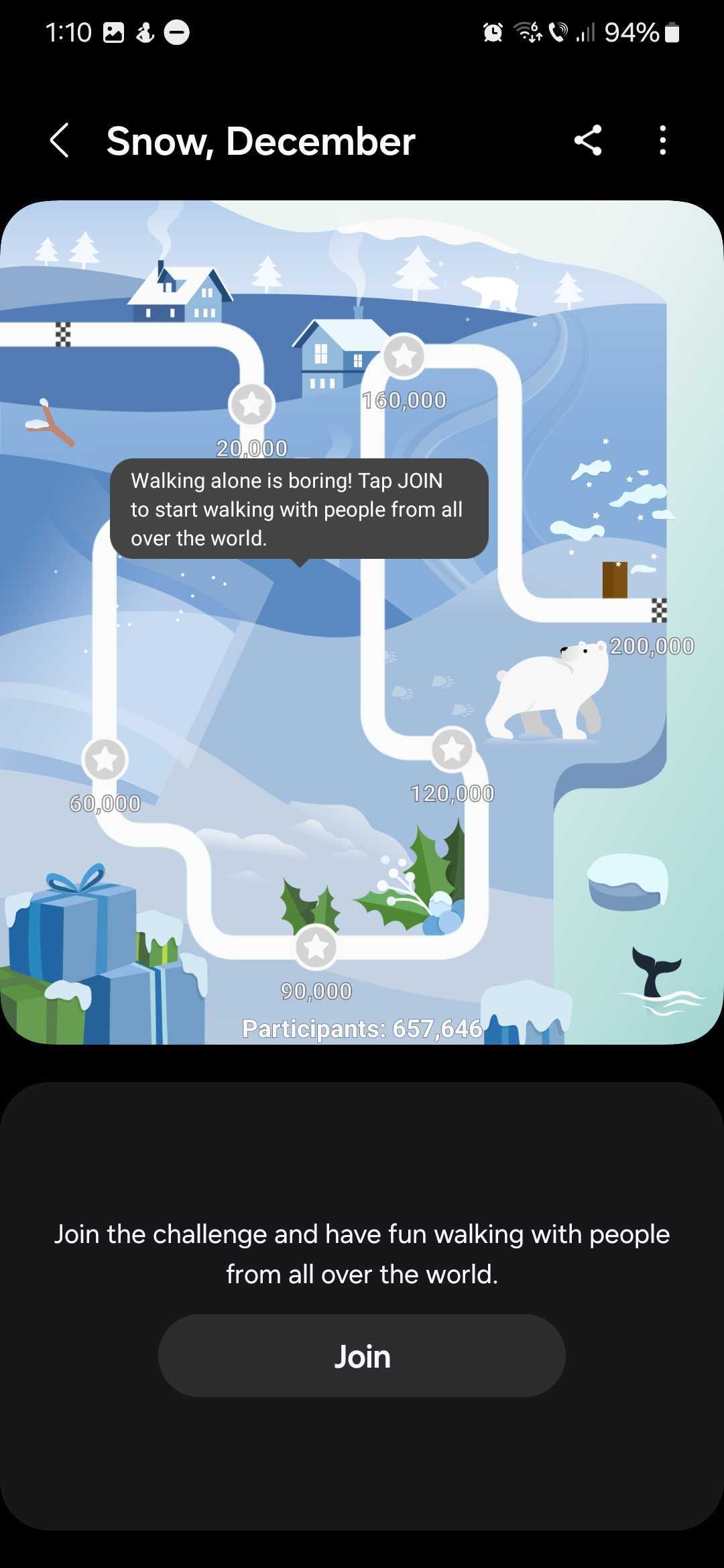**Caption:**

A screenshot of a smartphone display at 1:10, with several icons on the top left and a battery indicator showing 94% on the top right. An arrow pointing left is visible along with a label "Snow, December" in white font on a black background. On the top right, there are share and menu icons. Below, a full-width image with rounded corners occupies most of the screen. The image depicts a snowy game scene with a couple of houses lining a winding road. In the bottom left corner, there are several snow-covered gift boxes, while in the bottom right corner, a whale's tail is seen emerging from water. Near the middle, there appears to be a white dog or a polar bear. The road, marked by several stars denoting scores (200,000, 160,000, 120,000, etc.), leads players in a challenge to join and enjoy walking with others worldwide. The primary message encourages participation with the phrase "Join the challenge and have fun walking with people from all over the world, join."